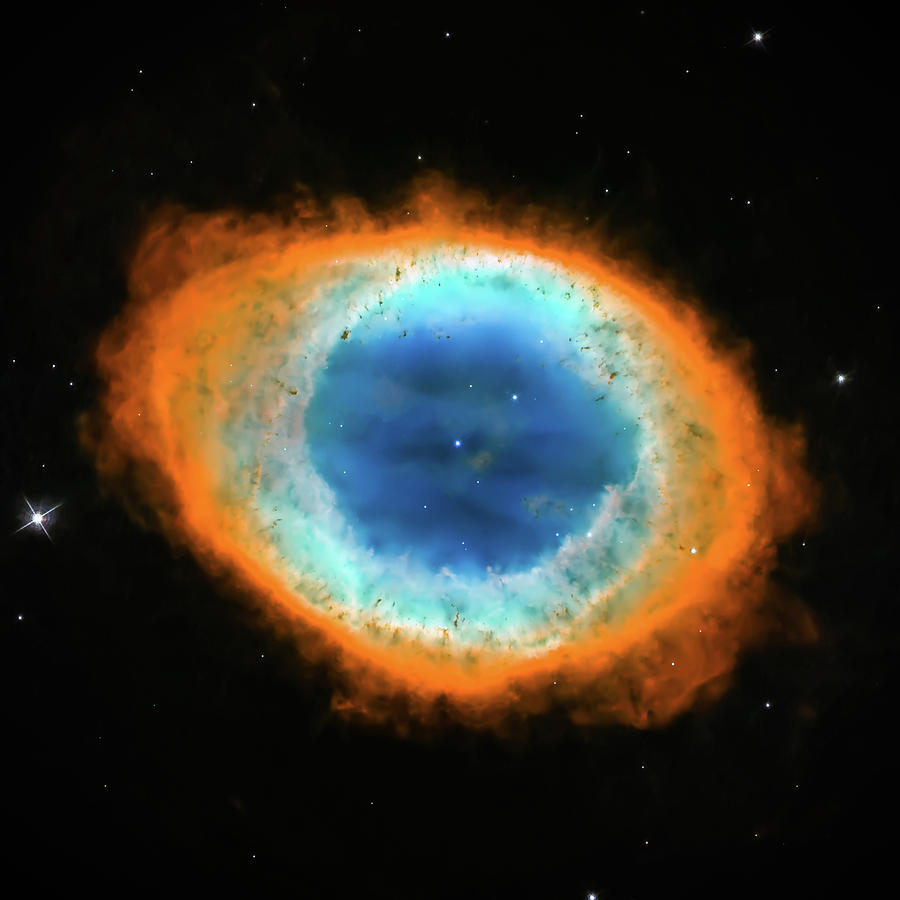This vivid photograph, likely taken by the Hubble Space Telescope, captures the mesmerizing Ring Nebula set against a jet-black star field peppered with individual stars. Dominating the image, the nebula dazzles with a spectrum of colors: a deep blue center, surrounded by an aqua blue ring, which transitions to a fiery, wispy orange outer layer that stretches almost to the edges of the photo. The nebula's shape resembles an eye, with an almost perfectly rounded central blue circle and an oblong, egg-like orange perimeter tilting slightly to the left. Strewn throughout the nebula are various stars, including some notably bright ones that exhibit cross-shaped artifacts, likely due to telescope mirror supports. Dark streaks add texture and depth to the image, highlighting the nebula's intricate structure and dynamic appearance.